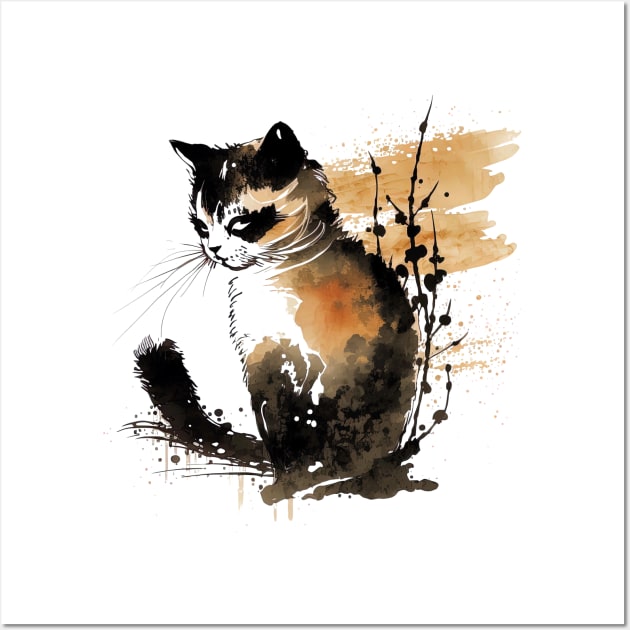This impressionistic painting depicts a ragdoll cat sitting upright on a white background. The cat has a distinct coat of various colors, including white, black, tan, brown, and a reddish-orange hue. Its chest and most of its face are primarily white, while the back, sides, paws, and tail are adorned with a mix of black, brown, and gray. The cat’s ears are pointed and dark, and its eyes are very dark and slightly slanted, contributing to a cartoon-like appearance. It has long, black and white whiskers, with a white mouth and lower face framed by black accents around the eyes.

The cat is oriented in a profile-like angle, gazing slightly to its right. Its entirely black tail is visible on the left side of the image. Behind the cat, there is a reed-like plant and assorted dark branches, adding depth to the scene. The backdrop contains light brown paint spatters, drip markings, and circular designs, introducing a dynamic, artistic texture to the composition. An orange smear also enhances the background, complementing the cat's reddish-orange patches and creating a harmonious visual effect.